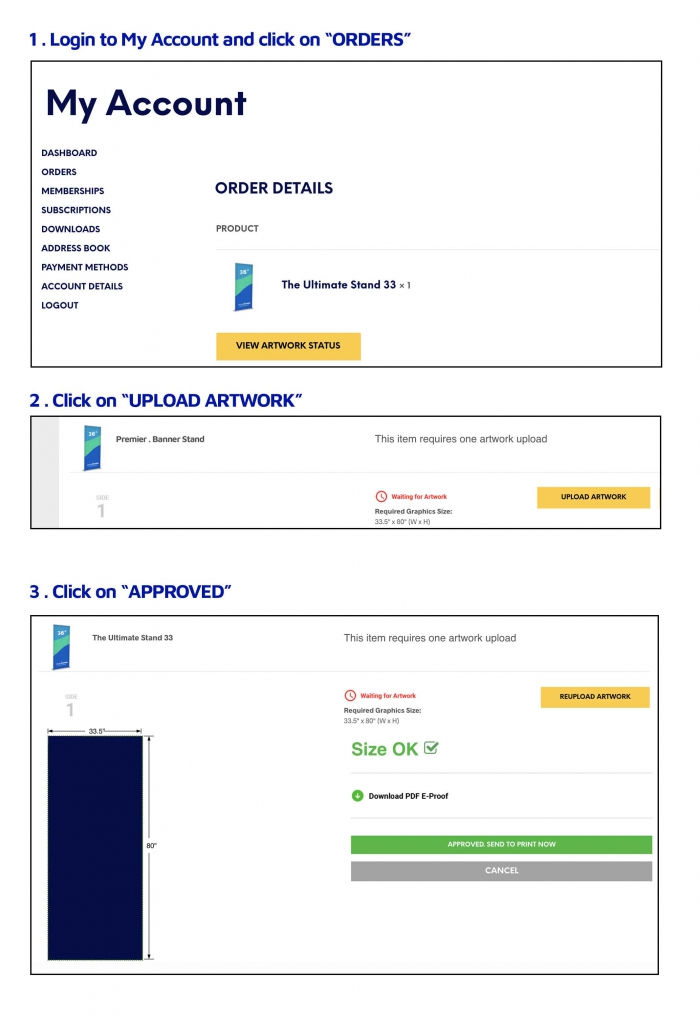This image depicts a detailed user interface from an online printing service's account dashboard. At the top of the screen, there is a login area. Once logged in, the dashboard presents various options including orders, membership, subscriptions, downloads, address book, payment methods, account details, and logout.

Alongside the dashboard options, the interface shows order details, specifics about products, and a rectangular widget that directs users to "view artwork site." There is a button labeled "upload artwork" accompanied by instructions indicating that the site requires one artwork upload. A yellow square prominently displays "upload artwork."

There are comprehensive details about the required graphics' size, and a button marked "approved" is present. The top left section of the screen reiterates the requirement for one artwork upload and its associated size. A green checkmark appears next to the text "download PDF e-proof," indicating a finalized review process. 

A large blue rectangle with arrows illustrates the measurement sizes—33.5 inches by 30 inches—suggesting the print dimensions. The screen seems to be part of a website dedicated to facilitating the upload and printing of artwork, possibly for banners or stands.

The entire setup hints at an organized workflow for users to upload, approve, and send their artwork to print, complete with visual aids to ensure accuracy in the artwork dimensions.